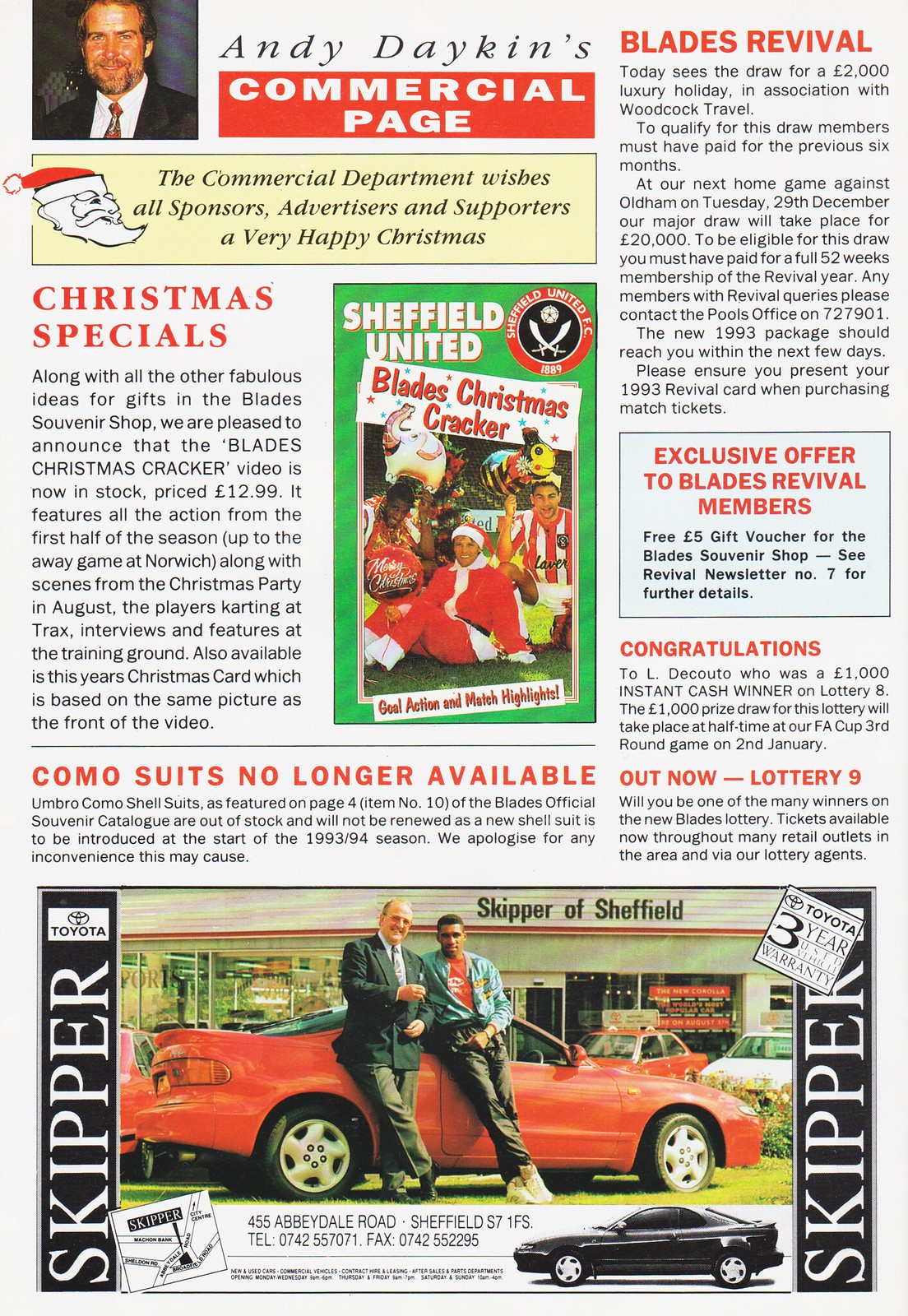This appears to be a detailed scan of a colorful magazine page, potentially from the 80s or 90s. In the top left corner, there is a photograph of a man in a business suit, identified as Andy Dakin, accompanied by the title "Andy Dakin's Commercial Page". To the right of the photo, a message extends festive greetings: "The commercial department wishes all sponsors, advertisers, and supporters a very happy Christmas." Below this, a yellow box with a Santa head drawing reinforces the Christmas theme. The page is filled with various articles titled in red, such as "Christmas Specials," "Como Suits No Longer Available," "Blades Revival," "Exclusive Offer to Blades Revival Members," "Congratulations," and "Out Now Lottery Number Nine." A smaller inset shows another magazine issue featuring the Sheffield United Blades Christmas Cracker with goal action and match highlights. At the bottom of the page, there's an advertisement for "Skipper of Sheffield," showcasing an older caucasian man and a younger African-American man standing in front of a red sports car, implying a dealership context with the word "Skipper" and "Toyota" prominently displayed.